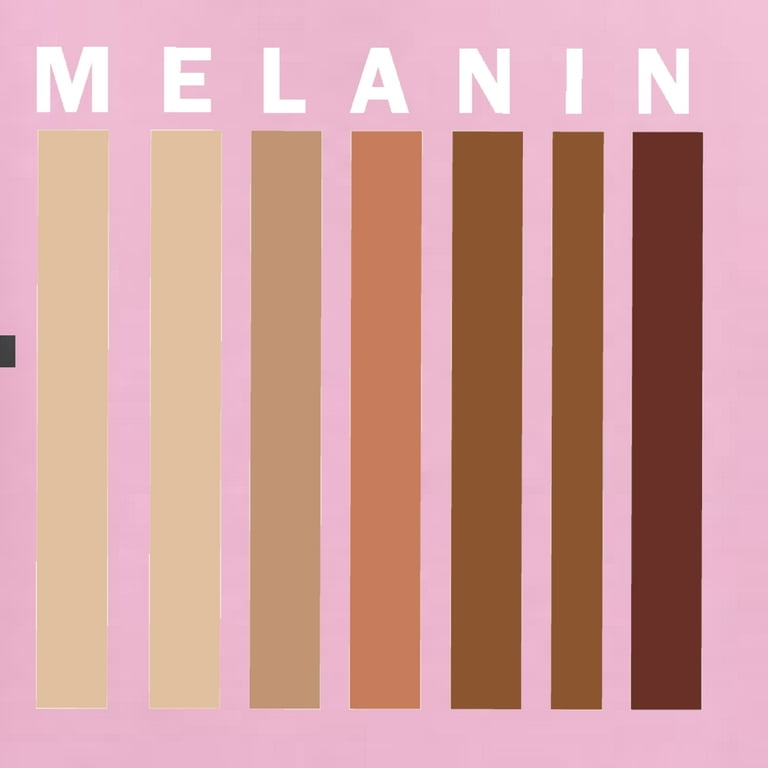The image features a light pink background with the word "MELANIN" displayed prominently at the top in all caps, white font. Below each of the seven letters is a vertical rectangle, each in a different shade, suggesting various skin tones. These rectangles range from light tan on the far left to a dark reddish-brown on the far right. Specifically, the colors transition from a light beige, to a moderate tan, to an orangish brown, followed by a darker tan, a light sepia, a darker brown, and finally, a dark brick brown. Additionally, there's a small black rectangle located in the middle on the left side of the image. The arrangement and color gradient emphasize the diversity of melanin in skin tones.